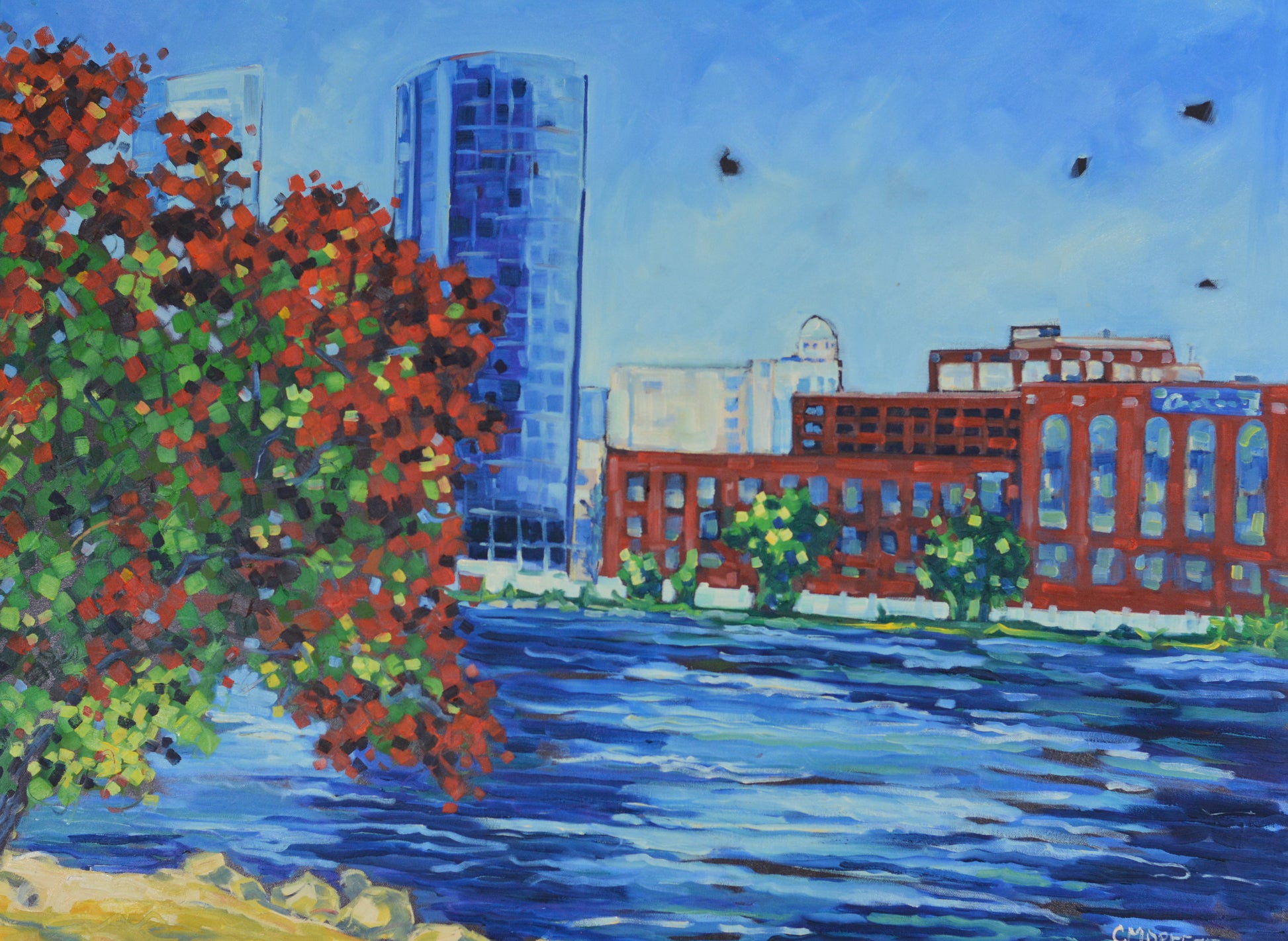This image portrays an impressionistic watercolor painting of an urban cityscape adjacent to a body of water, possibly a canal or small lake. The scene features various shades of blue, prominently displayed in the water and the sky, which has patches of white suggesting clouds. On the left, there's a bush or tree with leaves depicted as colorful splotches—green, red, yellow, and black—extending over the water. The middle-left side of the image showcases a blue skyscraper, while the right side includes smaller multi-storied buildings in white and red. The horizon is marked by a distinct area of yellow land at the bottom left, atop which the colorful bush is growing. Black bird silhouettes can be seen flying against the blue sky, particularly in the upper right corner. The painting uses an array of squares and splotches to create this vibrant urban landscape, blending impressionistic and pointillism-like techniques.